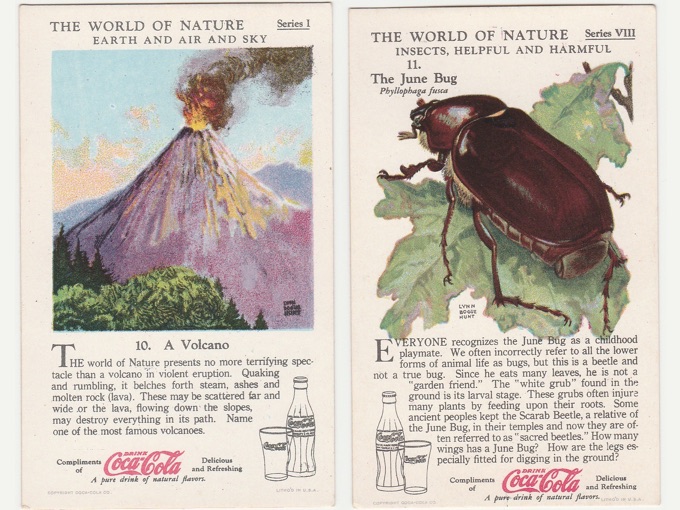This image features two vintage educational trading cards, sponsored by Coca-Cola, each adorned with the iconic Coke bottle and glass illustrations, along with the slogan "Compliments of Coca-Cola, a pure drink of natural flavors, delicious and refreshing." The cards appear aged, printed in grainy colored illustrations, suggesting an early to mid-20th century origin. 

On the left is a card from "The World of Nature, Series I, Earth and Air and Sky," titled "A Volcano." Its color illustration depicts a dramatic volcanic eruption with billowing smoke, vibrant red lava, a background mountain, a blue sky, and a foreground with tan clouds and trees. The text vividly describes the terrifying spectacle of a volcanic eruption, highlighting its destructive power with lava and debris.

The card on the right belongs to "The World of Nature, Series VIII, Insects, Helpful and Harmful," showcasing "The June Bug." The illustration features a June Bug, positioned on an oak leaf, seen from a rear, angled view. The accompanying text differentiates the June Bug from true bugs, notes its role in harming plants by feeding on leaves and roots, and touches on historical aspects of its scarab beetle relatives being considered sacred. Both cards incorporate questions to engage further thinking about the subjects.

Overall, these educational cards with their nostalgic art and informative blurbs illustrate the rich and intriguing world of nature, cleverly sponsored by Coca-Cola.